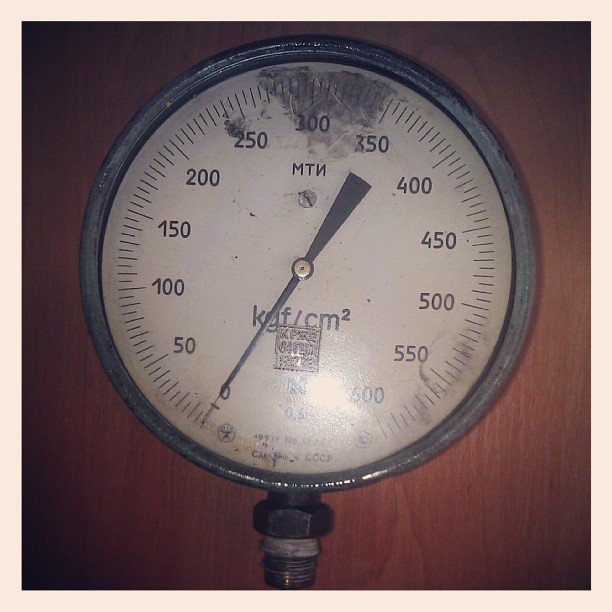This image depicts a pressure gauge set on a wooden desk or table. The gauge has a black metallic casing and a screw securing it at the base. It is illuminated from above by a bright light, which causes a noticeable glare on the gauge's surface. The dial features a singular needle currently pointing to zero, positioned at the seven o'clock mark on the gauge’s face. 

The scale extends in a clockwise direction, marked in increments of 50 from zero to 600, with the maximum value located at the five o'clock position. The measurement unit on the dial is "kgf/cm²". At the top of the dial, there are Cyrillic letters, possibly indicating that the gauge is labeled in Russian. Additionally, the top part of the gauge's casing is scuffed, obscuring the numbers 300 and 350.